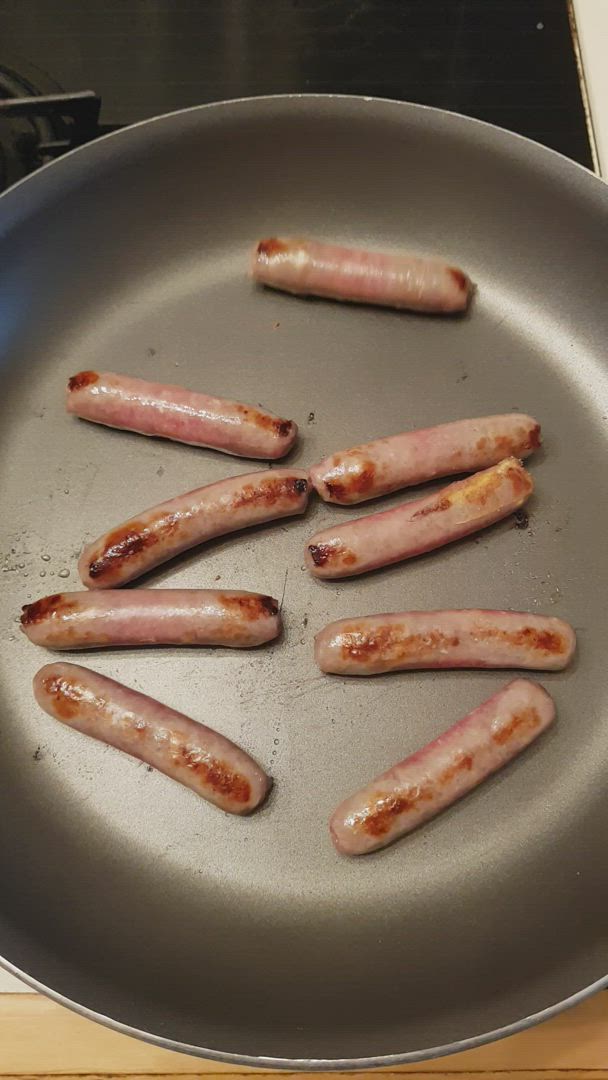A detailed overhead shot shows an aluminum skillet placed on a black stove grate. The skillet, silver in color, holds nine sausage links aligned horizontally, with four on each side and one near the top, slightly apart from the rest. These sausages are pinkish with hints of browning, particularly at the tips and edges, indicating they are being cooked. The background features a black stove ridge and a glimpse of a light blonde wooden table at the bottom edge of the image. The sausages, albeit pink, exhibit grill marks and some browning, suggesting varying stages of doneness.